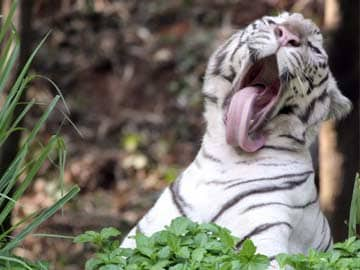This photograph captures a white tiger mid-yawn, prominently displaying his long pink tongue extending to the base of his neck. The tiger, adorned with striking black stripes and sporting a pink nose, sits amidst a backdrop of green grasses and surrounding foliage. His head tilts slightly to the left, eyes squinted, and whiskers vividly visible. In the background, partially blurred, are hints of brown and green leaves, coupled with some tall, slender trees on the right side. The rectangular image highlights the relaxed posture of the tiger, creating a tranquil yet striking outdoor scene.